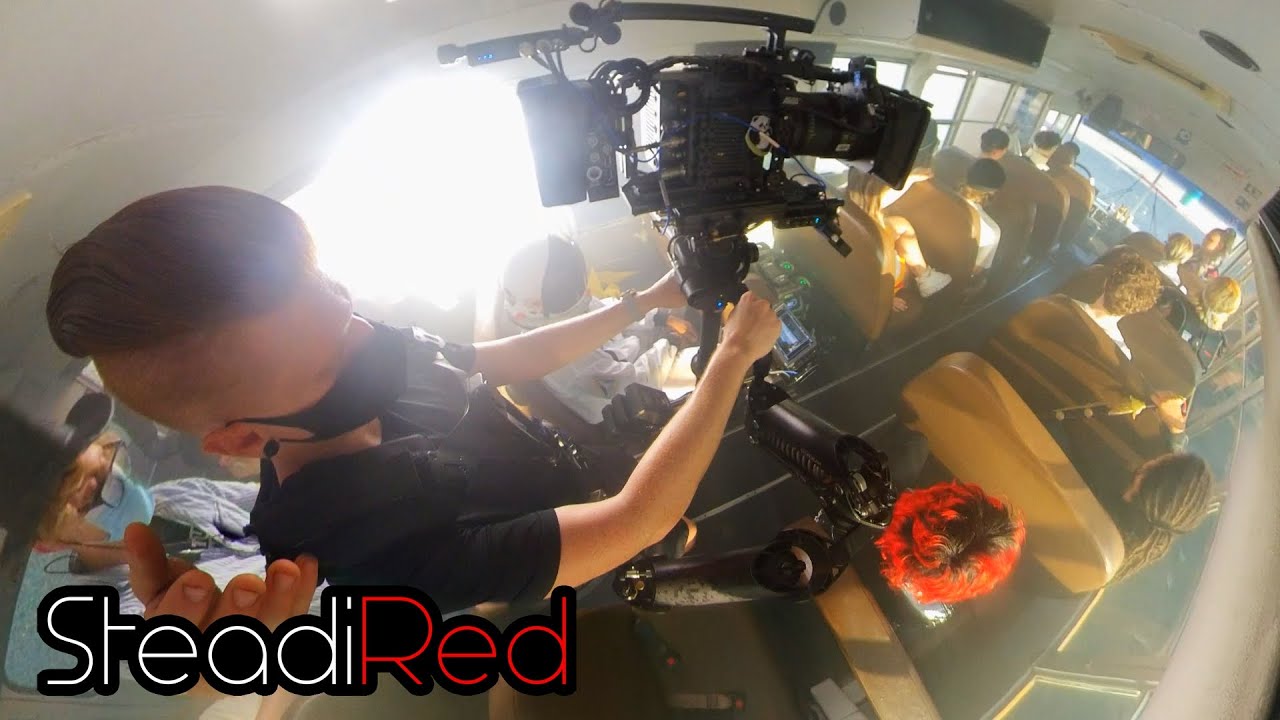The image is a color landscape photograph capturing an interior scene of a bus filled with passengers. At the lower left corner, a young camera operator is prominently featured. He is wearing a short-sleeved black t-shirt and a black face mask, with his ears adorned with large black gauges. His hair is shaved on the sides with the top longer. He is equipped with a black canvas rig on his chest, which supports a large black movie camera via a significant black metallic arm. The man appears focused, with his hands extended to adjust the camera. Behind him, another man, wearing a light blue shirt, a black top hat, and a blue face mask, can be seen. 

The bus itself has white walls and a roof, along with numerous glass windows on both sides. Inside, most of the tan-colored bench-like seats are occupied. In the bottom right corner of the photo, a passenger with hair dyed with red highlights is visible, adding a burst of color to the scene. Additionally, there is text in the lower left corner reading "SteadiRed" in a combination of white and red colors. The viewpoint of the photograph is slightly elevated, offering a comprehensive view of this busy, controlled environment where the driver can be seen in the far right upper corner among the glass windows.